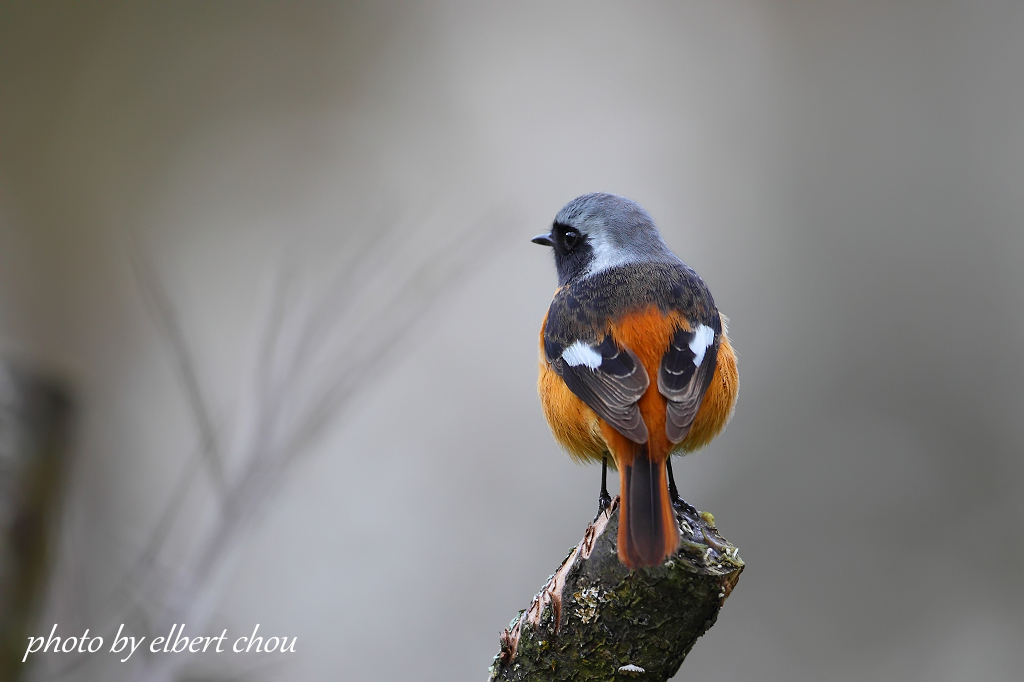This color photograph captures a small, vibrant bird perched at the end of a dark brown branch in the close-up foreground. The bird, occupying the lower center-right of the image, is facing slightly to the left, showcasing the intricate details of its plumage. Its head is gray with a distinct black ring around its beady black eye and a black beak. A hint of white can be seen amidst the gray and black feathers. The bird's upper back, wings, and parts of its tail display a mix of brown, black, and white feathers, while its chest, underbelly, and the majority of its tail are a striking orange color. The background, largely blurred in a wash of gray with faint, shadowy branches off to the left, ensures full attention remains on the colorful bird. Its black legs grasp tightly onto the branch. Notably, the photograph credits "Photo by Elbert Chou" in the bottom left corner, adding authenticity and recognition to this beautifully captured moment.